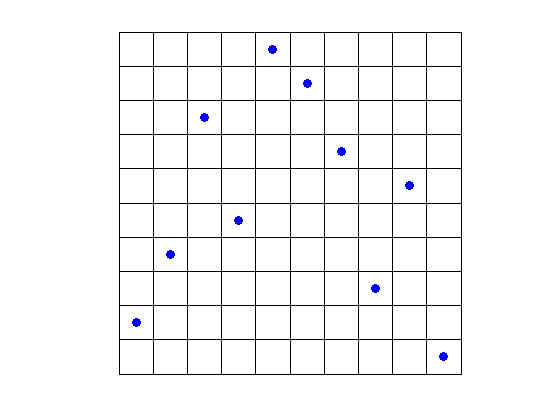The image depicts a computer-generated or hand-drawn 10 by 10 grid composed of 100 individual white squares outlined by black lines, forming an overall square shape on a white background. Within this grid, there are ten unique squares, each featuring a single purplish-blue dot located in the center. Each of the ten dots occupies a distinct row and a distinct column, ensuring no two dots share the same row or column. The blue dots are dispersed across the grid, and while their placement appears randomized, the unique positioning in separate rows and columns suggests a deliberate arrangement. The color palette of the image is limited to black, white, and blue, emphasizing the simplicity and precision of the grid and the marked squares.